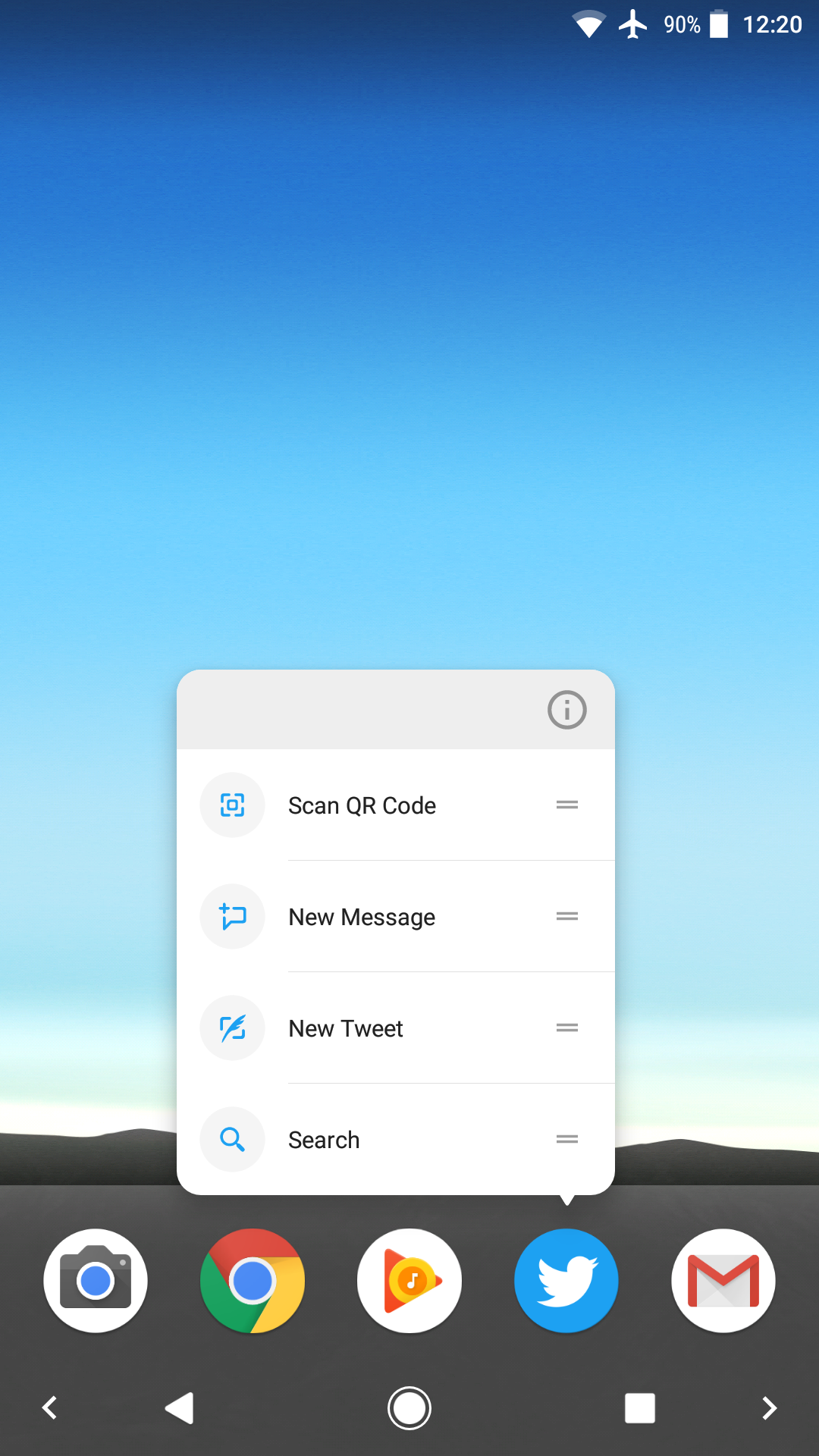This is a detailed screenshot of a smartphone home screen, featuring a visually striking background of a cartoon-like mountain range under a dynamic blue sky. The gradient sky transitions from a deep blue at the top, gradually lightening as it approaches the peaks of the mountains, culminating in an almost white hue where it meets the jagged, snow-capped summits. At the bottom of the screen, there's a wide brown horizontal border, home to several important app icons: Camera, Chrome, YouTube Music, Twitter, and Gmail.

Dominating the center lower half of the screen is a white pop-up box, partially obscuring the Twitter icon. This pop-up box has a subtle gray border at its top edge and is white throughout the rest. It provides quick access to several actions within the Twitter app, listing options for "Scan QR Code," "New Message," "New Tweet," and "Search." The overall layout is both functional and aesthetically pleasing, providing a snapshot of a user's organized digital life against a serene and picturesque backdrop.